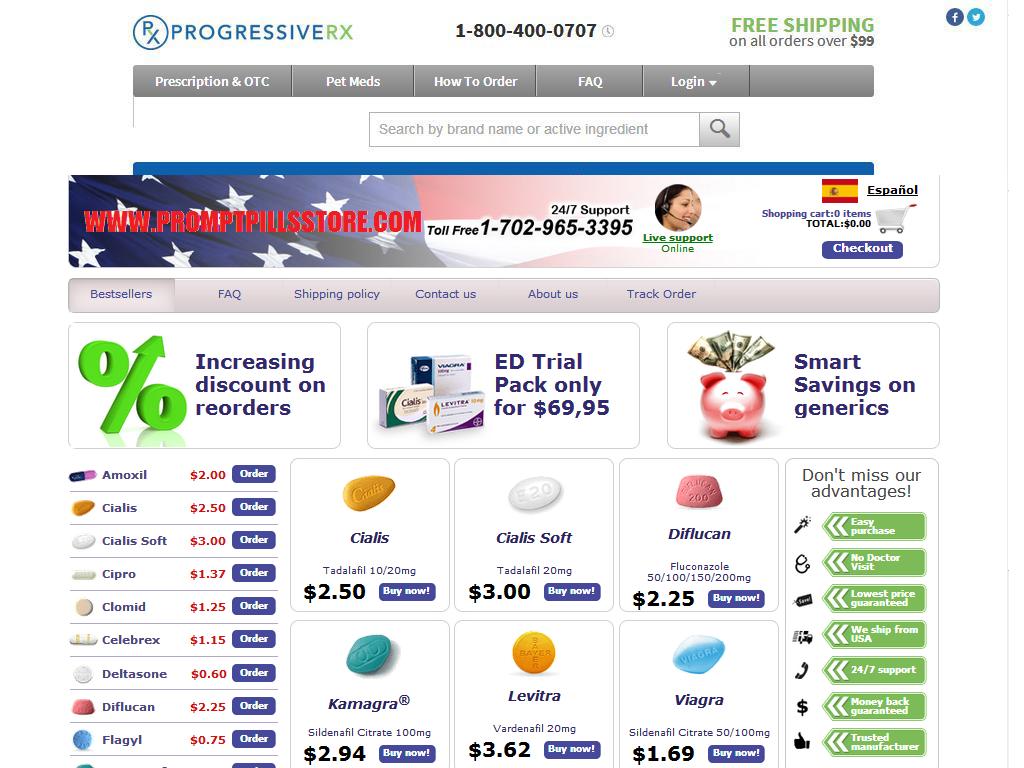At the top of the website, the banner prominently displays the text "Progressive Rx" in bold, bright green letters. Accompanying the text is a stylized "Rx" symbol; the "R" features an elongated leg that extends outward at an angle, intersecting with the "X" overlaid on it. This symbol is encircled in a teal-blue circle. Below this, in the center, an 800 number—1-800-400-0707—is clearly visible.

To the right, there's an enticing offer stating, "Free shipping on all orders over $99." Below this information, a gray toolbar with white font provides links to essential site sections: "Prescriptions and OTC" on the left, followed by "Pet Meds," "How to Order," "FAQs," and a "Log In" option with a dropdown menu. Adjacent to this toolbar is a user-friendly search bar that allows users to search by brand name or active ingredient.

A blue line separates the header from the main content. Just below this line, a prominent banner in large red font reads "www.promptpillsstore.com." Underneath this banner, another section features a photo of a flag and important contact information: "Toll-Free 1-702-696-5339." It also highlights "24/7 Support" and "Live Support Online" in green, accompanied by an icon of a woman wearing a headset, and includes the option for "Espanol" with a corresponding flag.

At the top right corner, there's a clear display of the shopping cart status: "0 items" with a total of "$0." The shopping cart icon is visibly placed here along with a blue "Checkout" button in white text, ensuring easy navigation for completing purchases.